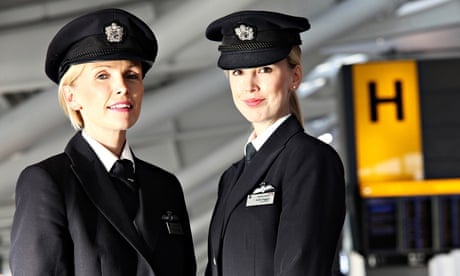The image depicts two presumed female pilots in their early 30s, captured from the lower chest up. Both women are Caucasian and dressed in matching pilot uniforms, consisting of black hats with seals on the front, black dress coats, black ties, and white undershirts. The pilot on the left is slightly older with short blonde hair pulled back, facing the camera directly and smiling with her mouth slightly open. The younger pilot on the right has long blonde hair, her body turned towards the eight o'clock position with her head tilted towards the camera, also smiling. They both have pilot wings visible on their left chest. In the background, to the right, there is a yellow conveyor machine marked with the letter "H," as well as white pipes on the ceiling and a gray structure, possibly a building or machinery.